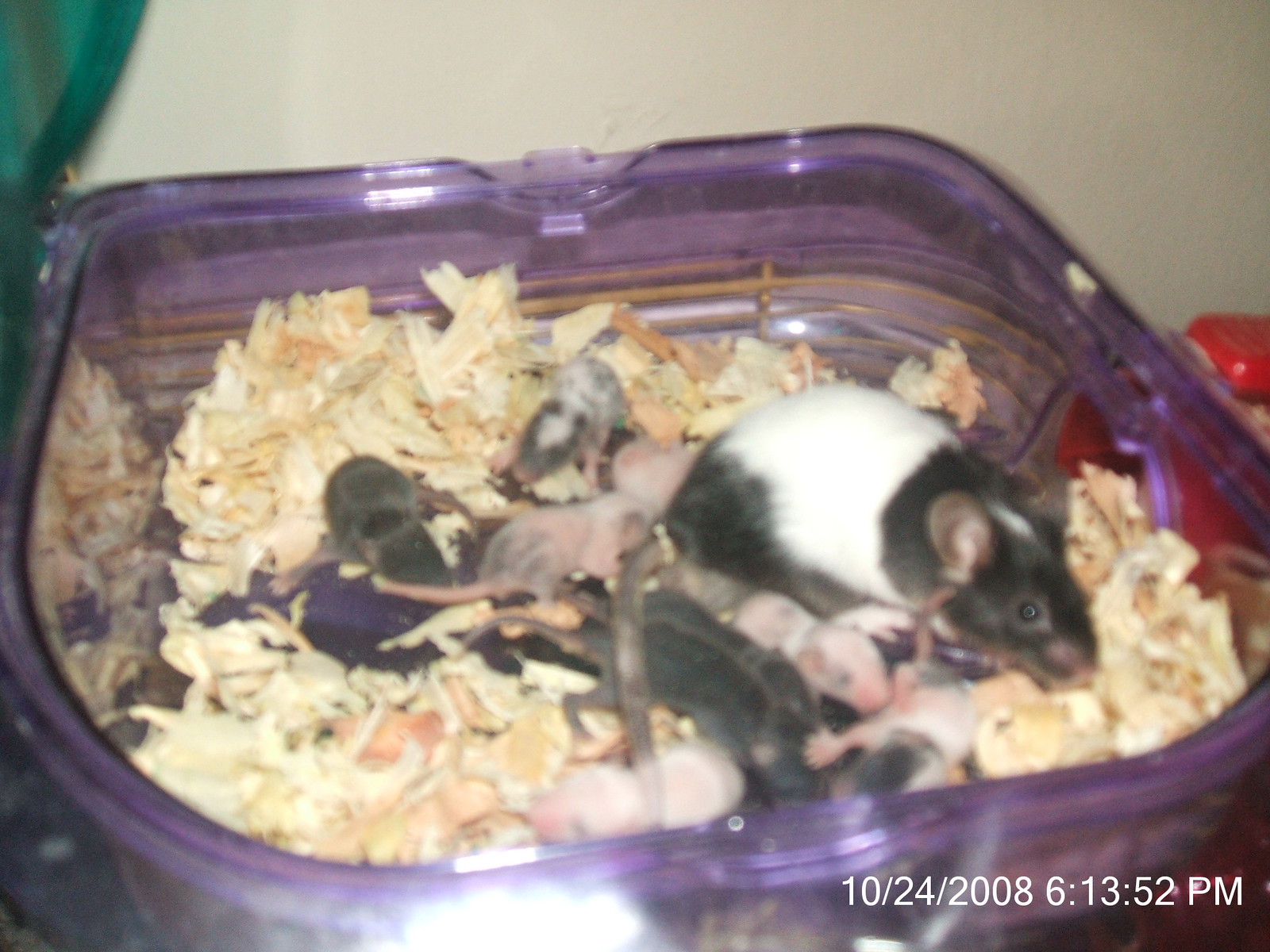The image captures a color snapshot of a mother mouse and her newborn babies inside a translucent purple plastic Tupperware container lined with wood shavings. The container, square in shape, sits on a white table or shelf against a tan-colored wall. The background includes a red object on the right and possibly a green curtain to the left. The mother mouse, which has distinct black and white markings, is positioned on the right side of the container, slightly turned to the right. She is accompanied by approximately five to nine baby mice, some of which have peach or flesh-colored skin, while others possess short black fur. The mice are variously sprawled across the wood chip bedding. The image, distinguished by its bright lighting and glare, features a timestamp—10-24-2008 6:13:52 PM—clearly visible in white text in the bottom right corner.